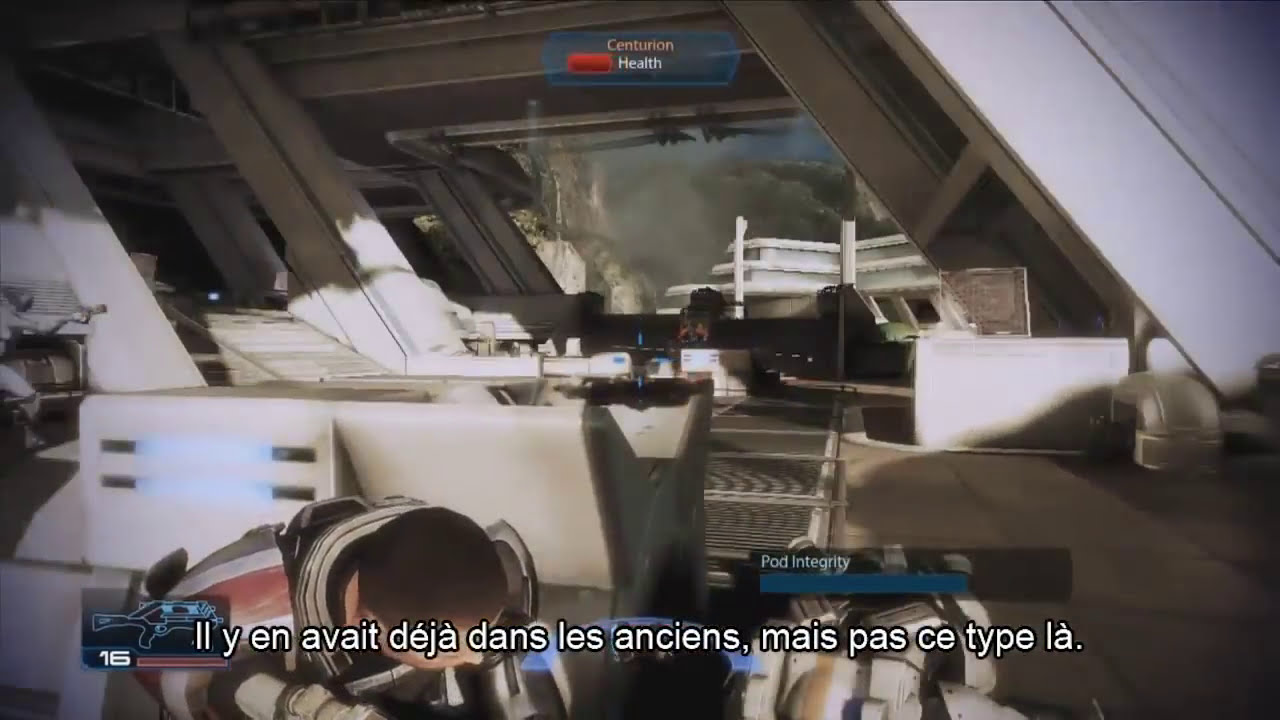This detailed screenshot from a three-dimensional French video game depicts an industrial, cluttered environment, possibly the interior of a spaceship or industrial facility, characterized by metal structures with slanted columns and overhead passes. The view is from a first-person perspective, suggesting the player is inside the structure. At the top center of the screen, the word "Centurion" is visible in red lettering, with a corresponding "Health" indicator and a quarter-full red health bar. The lower left corner displays an image of a gun, the number 16 indicating the ammo count, and a full red bar labeled "Pod Integrity," which is three-fourths full. French caption text at the bottom reads, "il y en avait déjà dans les anciennes mais pas ce type là," suggesting a context or narrative for the scene. The area also includes items like rails, bars, desks, and possibly a space suit or other equipment scattered in a jumbled heap, enhancing the detailed, industrial aesthetic of the setting.